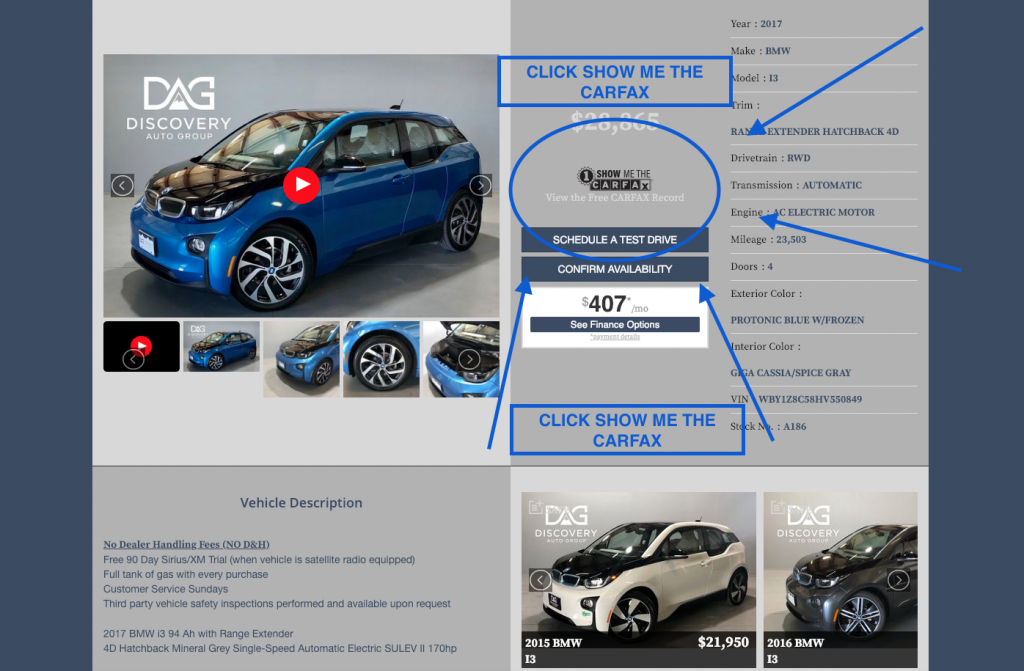The image depicts a detailed page on an automotive website, specifically for the Discovery Auto Group (DAG). Dominating the top left corner is a blue BMW, which features a YouTube-style play button indicating that a video, likely showcasing the car’s exterior and interior details, is available. Below the video, close-up screenshots of the vehicle are displayed, providing additional visuals.

Immediately beneath these images is a box containing a detailed vehicle description, which includes key specifications such as the year (2017), make (BMW), model (13), trim, drivetrain, transmission, engine details, mileage, number of doors, exterior color, interior color, VIN number, and stock number.

On the right-hand side, the vehicle's price is prominently displayed. There is also a blue circle with arrows pointing towards it, highlighting the option to "Show me the Carfax" twice, emphasizing the importance of the Carfax report for prospective buyers. The website further provides options to schedule a test drive, confirm availability, view finance options ($407 per month), and see additional pricing details.

Beneath the primary vehicle information, the site suggests two other BMW models for comparison: a 2015 BMW and a 2016 BMW, offering users the ability to browse similar vehicles.